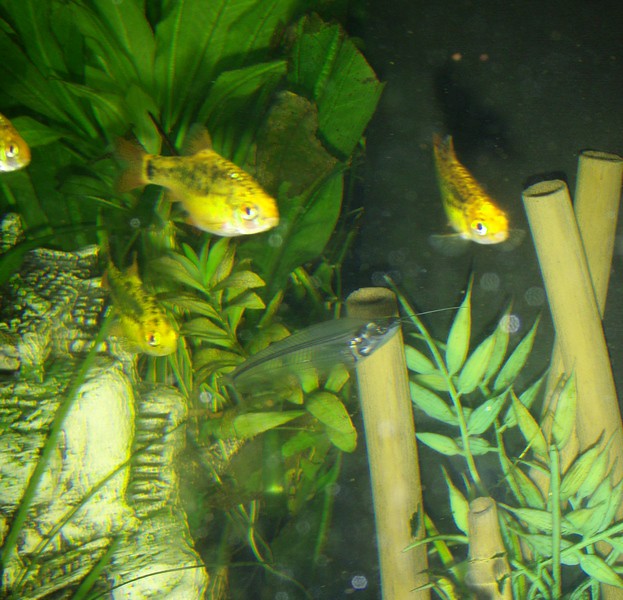The photo captures a captivating underwater scene within a fish tank, which exudes a dark, mysterious ambiance with its murky depths. The tank houses five distinct fish; four are goldfish-like, displaying a yellow-green hue with black spots, each equipped with slightly bulging eyes. The standout fifth fish resembles a miniature swordfish, semi-transparent with a black spine and a silvery-gray, spear-like nose, creating a striking contrast with the others.

The tank's bottom right corner is adorned with four decorative, light brownish-yellow bamboo tubes set amidst lush green plants. These bamboo shoots rise from the substrate, with one standing upright in the center, another laying low, and two crisscrossed on the right, accompanied by vibrant green foliage scattered throughout. The left side hosts additional green and yellow-tinged plants alongside white rocks streaked with green, adding to the tank's exotic aesthetic.

A stone structure, possibly resembling a small house or hut with a tiled roof and steps, adds an element of intrigue to the tank's elaborate setup. The backdrop is predominantly dark, particularly in the right corner, which heightens the mysterious feel of the scene. Conspicuous are two red spots that might resemble eyes, further contributing to the tank’s enigmatic atmosphere. The entire scene bathed in a dim greenish light, highlighting the abundant plant life and the unique inhabitants, creates a beautifully detailed, underwater paradise.